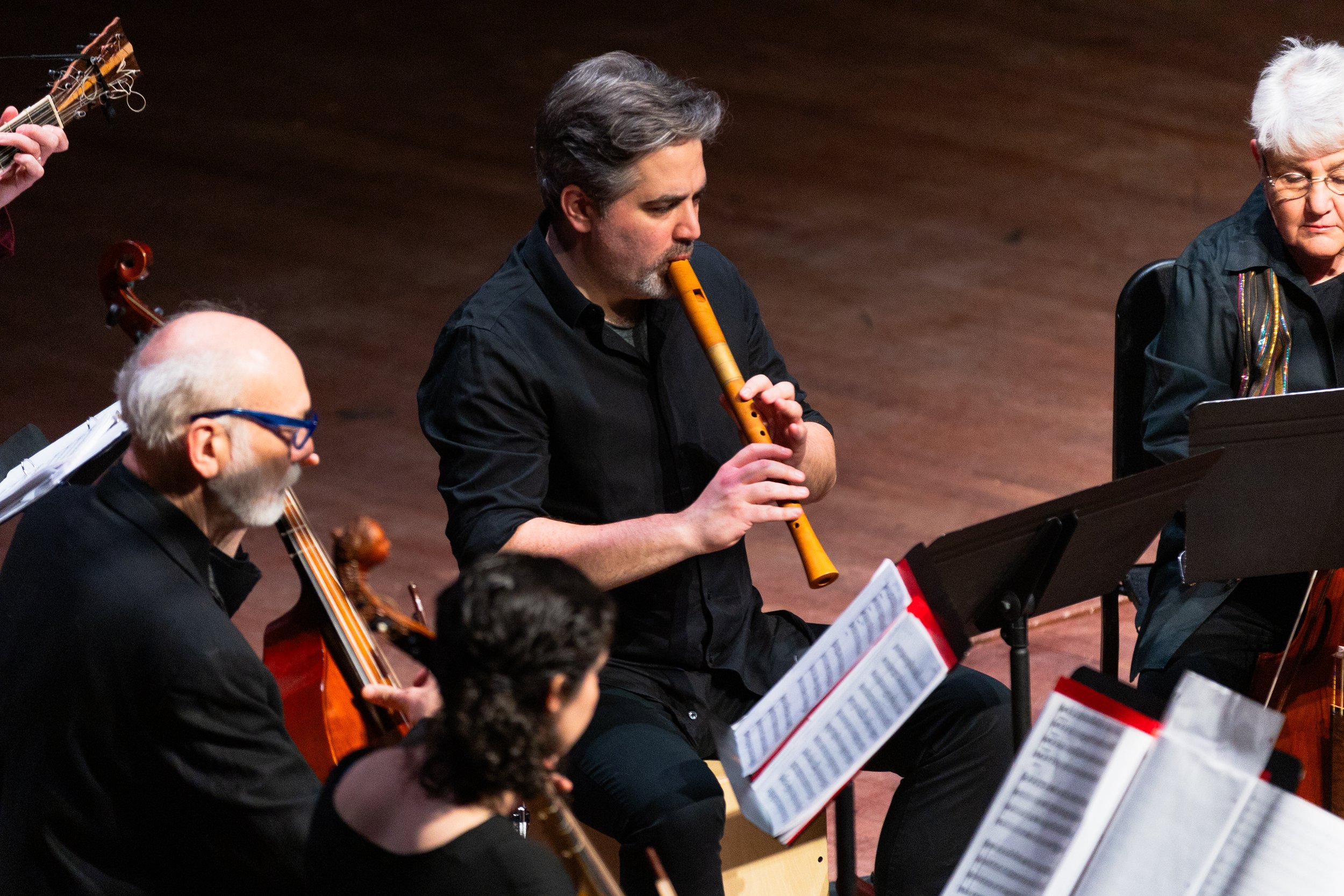This photograph depicts a section of an orchestra or band in mid-performance, focused primarily on a middle-aged man with dark, slightly graying hair. He is playing a yellow wind instrument, likely a wooden recorder, and is dressed in a long-sleeved, black shirt with the sleeves rolled up and black pants. Positioned in the center facing to the right, he is engrossed in his sheet music placed on a stand before him.

To his immediate left is an older, bald man with white hair, a short white beard, and striking blue eyeglasses, dressed in a black collared shirt. He is playing a large stringed instrument, presumably a cello, with his own sheet music stand in front of him.

In the foreground, there's a rear view of a female musician with dark, curly hair pulled back into a ponytail, also dressed in black. Her instrument isn't clearly visible.

On the far right, partially out of frame, is an elderly woman with white hair and thin glasses, adorned in a dark shirt featuring metallic ornamentation. She too is playing a stringed instrument, though only a small part of it is visible.

Additionally, the top left corner of the image captures the headstock of a guitar along with a hand forming a chord, suggesting another musician just out of the frame. Overall, the image captures a moment of focused, collective musicianship, with each performer intently engaged with their music.